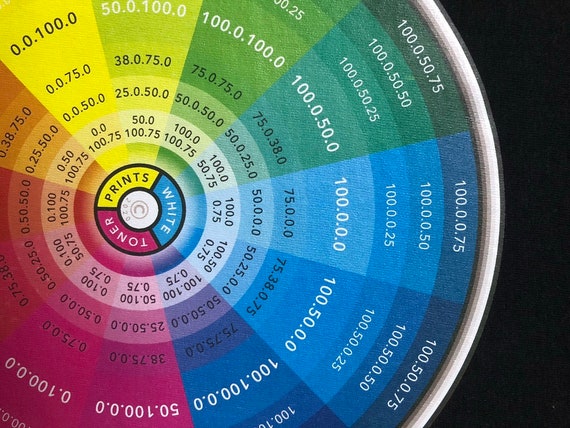This image showcases a vibrant, partially visible color wheel against a black background. The wheel, taking up three-quarters of the screen and positioned slightly off-center to the left, transitions from intense dark shades at the perimeter to lighter shades towards the center. Each wedge-shaped section of the wheel represents a color of the rainbow, including dark blue, light blue, green, yellow, orange, red, pink, magenta, and purple. Every section contains a unique number correlating to the specific shade. At the very center, the wheel is divided into three segments labeled "Prince" on a yellow background, "White" on a blue background, and "Toner" on a red background. The overall composition and labeled sections suggest an association with color grading, possibly used in photography or printing.